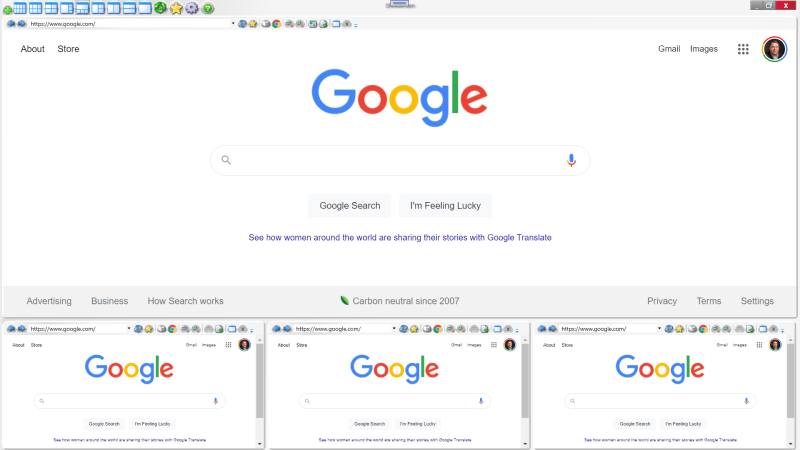This image captures a screenshot of a computer screen open to the Google homepage. Prominently displayed in the center are the iconic multicolored Google letters, directly above a search bar. At the far right end of the search bar is a microphone icon, indicating the option for voice search. Below the search bar, there are the familiar "Google Search" and "I'm Feeling Lucky" buttons. Further down, a message reads, "See how women around the world are sharing their stories with Google Translate."

At the bottom of the screenshot, there's a collage of three smaller images, each representing a view of the Google homepage. These additional images are aligned horizontally, with one on the left, one in the center, and one on the right. Each of these smaller images displays the URL "www.google.com" in the address bar. Notably, a profile picture of a man appears in the same position on all of these smaller images, including the main larger screenshot at the top, making a total of four identical profile pictures featured in the image.